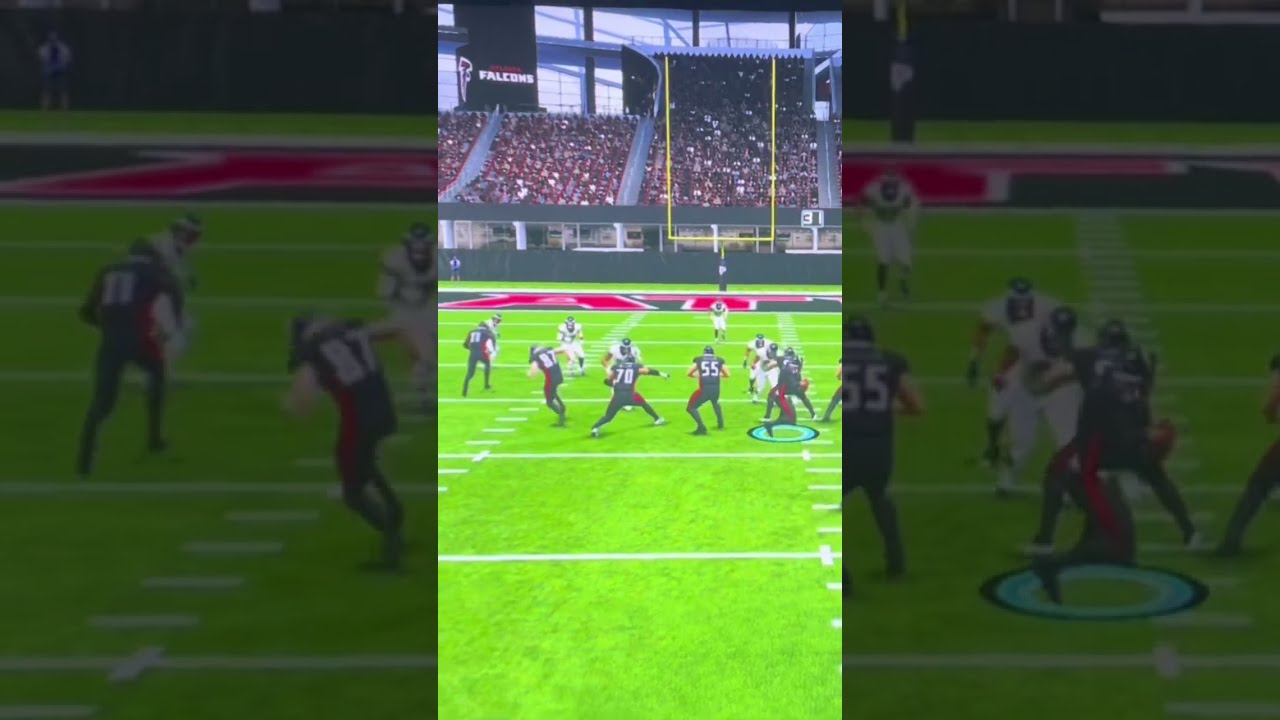In this detailed image of a video game, likely Madden, we see a football game taking place, presumably at Falcons Stadium. The image showcases a scene with the field, players, and audience. The playing field is green with white yard lines, highlighting the bold end zone painted in black with red letters spelling "Falcons." Amidst the view, the yellow goalpost stands prominently, and a large crowd fills the stands above, adding to the immersive sports atmosphere.

Central to the image are the players: one team clad in black and red jerseys, with numbers such as 11, 87, 70, and 55 standing out in the forefront, positioned around the 30-yard line. Their opposing team wears white uniforms. Notably, a blue circle beneath one player on the right suggests an active selection, indicating this is indeed an interactive game scenario.

The edges of the image are blurred, creating a visual focus on the central, vibrant action, which strongly hints that this might be a screenshot from a mobile device, possibly shared on platforms like Instagram or TikTok. In the upper-left corner, the text "Atlanta Falcons" is displayed, further cementing the setting of this engaging sports scene.